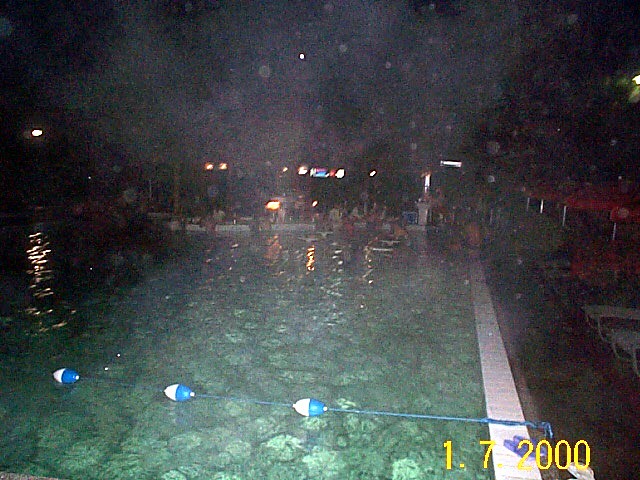The image depicts a swimming pool scene at night, heavily obscured and blurred, making details challenging to discern. The camera lens seems to be covered in smudges or water splashes, contributing to the overall indistinct quality. Despite this, the photograph shows a pool with a noticeable rope and floating separators indicating different depths. In the background, a gathering of people is visible, suggesting a swim-up bar might be present, though it's not entirely clear. The pool area is bordered in white, and to the right, there are several beach chairs and red or orange umbrellas set up. The scene is dimly lit, with some ground lights and light poles reflecting off the pool's greenish-tint water. The sky appears pitch black and includes some visual artifacts. In the bottom right corner, the image is stamped with the date "17-2000" in yellow.